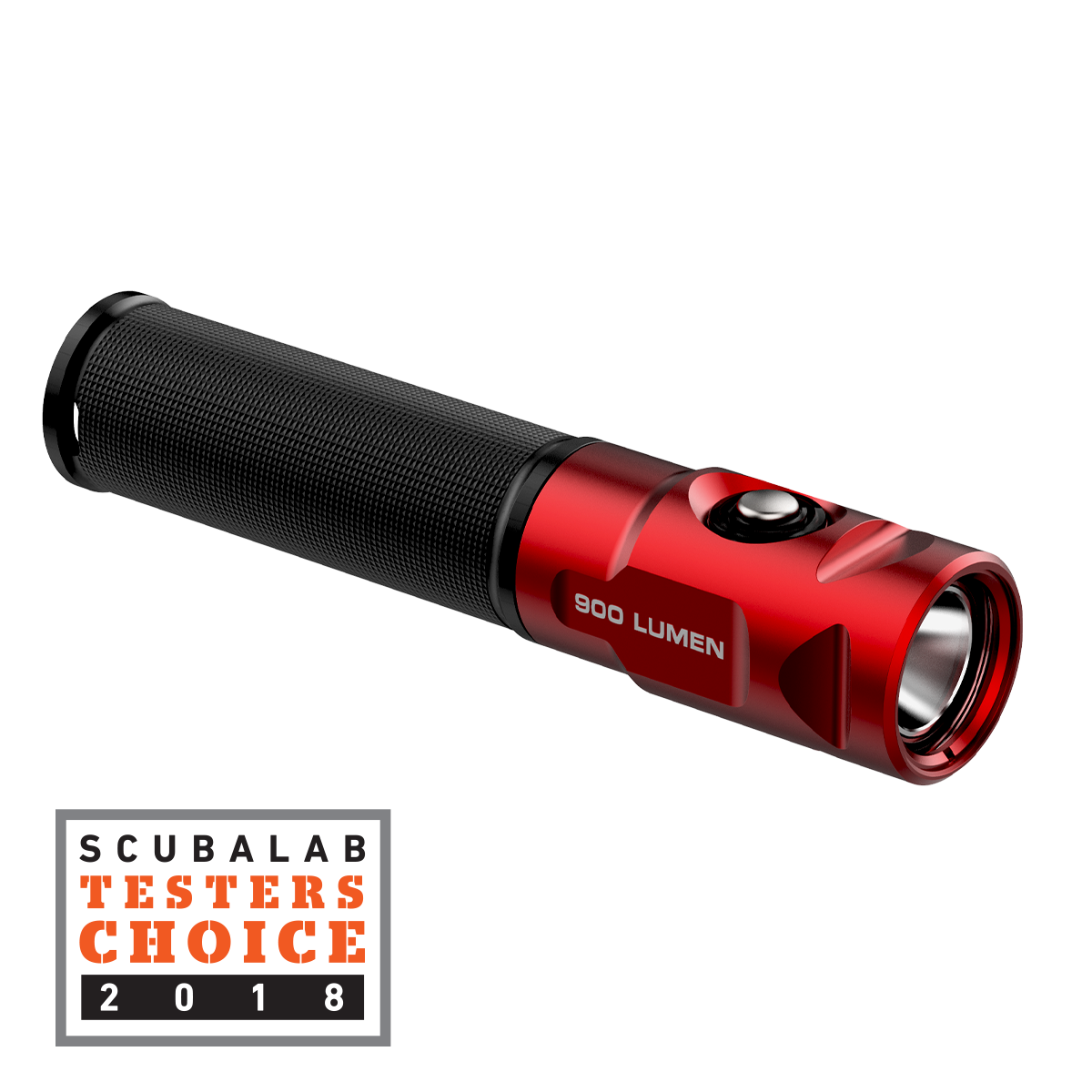The image features a photorealistic depiction of a durable, modern flashlight laid diagonally across a plain white background. The cylindrical-shaped flashlight is characterized by its two-tone design: the base where one would grip it is textured black, providing a non-slip hold, while the front end is made of red metal accentuated by several indents near the lens, which is silver since the flashlight is off. On its side, within another indent, the text "900 lumen" is prominently displayed in silver. A black and silver button is inset into the top section of the flashlight. In the bottom left corner of the image, there's a prominent graphic: a gray-outlined box containing the text "scuba lab" in black, followed by "TESTERS CHOICE 2018" in capitalized orange letters. This high-quality flashlight, described as compact enough to fit into a purse or backpack, showcases a robust design suitable for emergencies or outdoor activities.